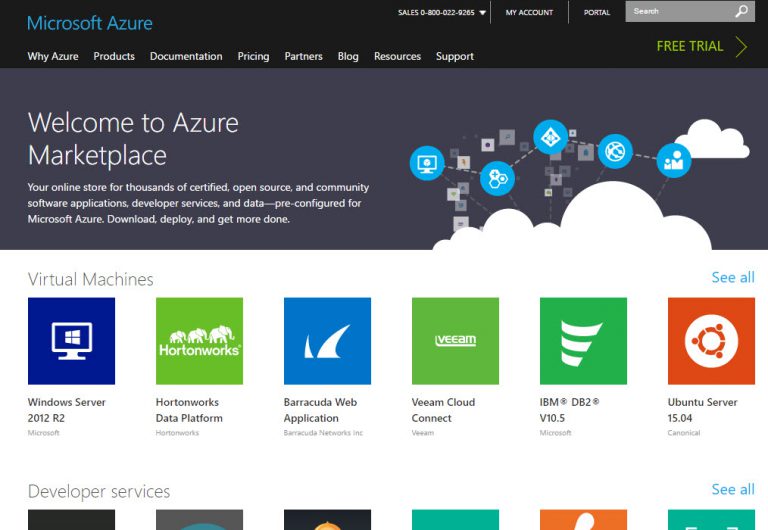A detailed screenshot from the Microsoft Azure application and Marketplace showcases the platform's interface and features. At the top, a black horizontal bar spans across the image, with the title "Microsoft Azure" in blue text situated at the upper-left corner. Directly beneath this title are subheadings for "Home," "Products," "Documentation," "Pricing," "Partners," "Blog," "Resources," and "Support."

In the upper-right corner, the interface provides contact options, including a sales number, an account settings link, a portal entry option, and a search bar. Below these options, a green hyperlink offers more information about obtaining a free trial.

Separated by a gray bar is a welcoming message that reads, "Welcome to Azure Marketplace," accompanied by a brief descriptive text. Adjacent to this message on the right is a graphic illustration featuring five interconnected blue circles with surrounding clouds, symbolizing cloud connectivity.

Beneath the gray bar, the interface displays several square application icons labeled as virtual machines, with an option to "See all" available to the user. The listed virtual machines include:

- Windows Server 2012
- Hortonworks Data Platform
- Barracuda Web Application
- Veeam Cloud Connect
- IBM DB2
- Ubuntu Server

Partially visible below these icons is a section titled "Developer Services," showcasing an additional five application icons.